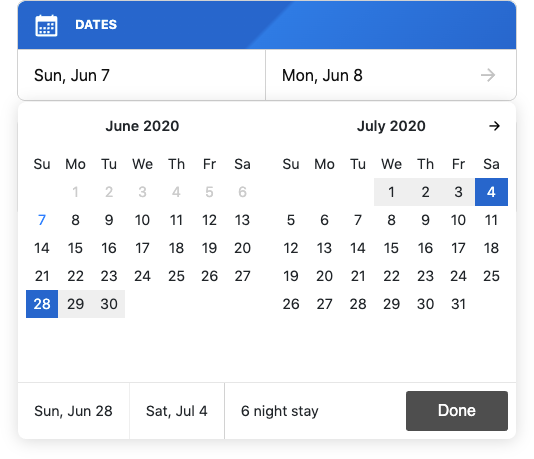The image depicts a digital calendar with a square aspect ratio and moderate quality, characterized by slight blurriness and fuzziness. The calendar features a primarily blue background, with a white calendar icon situated in the top left corner. Directly beneath the icon, the text "DATES" is displayed in all capital letters.

The main body of the calendar is divided into two prominent sections at the top. The left section displays the date "Sunday, June 7th," while the right section shows "Monday, June 8th," accompanied by a grey arrow pointing to the right, suggesting navigation to subsequent dates.

Further below, another divided section appears, with the left part marked as "June 2020." This section contains an array of days and their corresponding numbers, following a sequence for the days of the week abbreviated rather oddly as "S-U-M-O-T-U-W-E-T-H-R-F-S-A-E."

At the bottom of the image, additional date sections are present. On the bottom left, the date "Sunday, June 28th" is displayed, followed by "Saturday, June 29th."